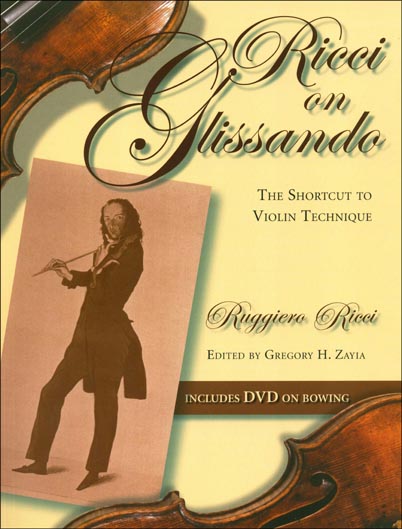The image appears to be the cover of an informational book on violin techniques. It has a yellowish background with photographs or drawings of violins partially visible in the top left and bottom right corners. Prominently featured in large black letters on the upper right corner is the title, "Ricci on Glissando." Below the title, in smaller black print, it says, "The Shortcut to Violin Technique." On the left side of the cover, there's an old-fashioned photograph of a violinist wearing a tuxedo with tails, appearing to be from the 1600s or 1700s. To the right of the image, in black letters, it reads, "Ruggiero Ricci," followed by "edited by Gregory H. Zaia." Below this, a small brown strip contains white text that indicates, "Includes DVD on Bowing."